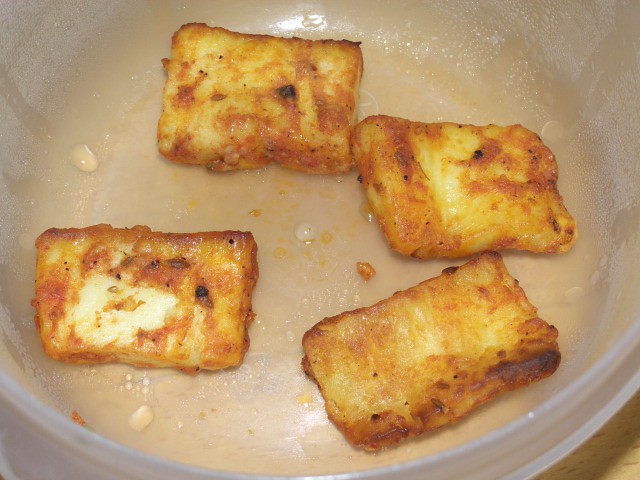The image is a close-up photograph of a bowl containing tater tots or possibly small hot pockets. The food pieces are square or rectangular, tinged with brown, yellow, and hints of red, likely due to cheese or sauce. The food appears greasy, with visible grease congregating at the center and seeping to the sides. The bowl, a plain circular plastic container, shows signs of moisture and perspiration, especially noticeable at the bottom left and right, suggesting it had been microwaved. The bowl is partly cropped out at the top and bottom edges of the image, highlighting the food's details and the bowl's plastic lining. The food pieces, four in total, remain whole and unbitten, indicating they haven't been eaten yet, possibly having just been reheated.